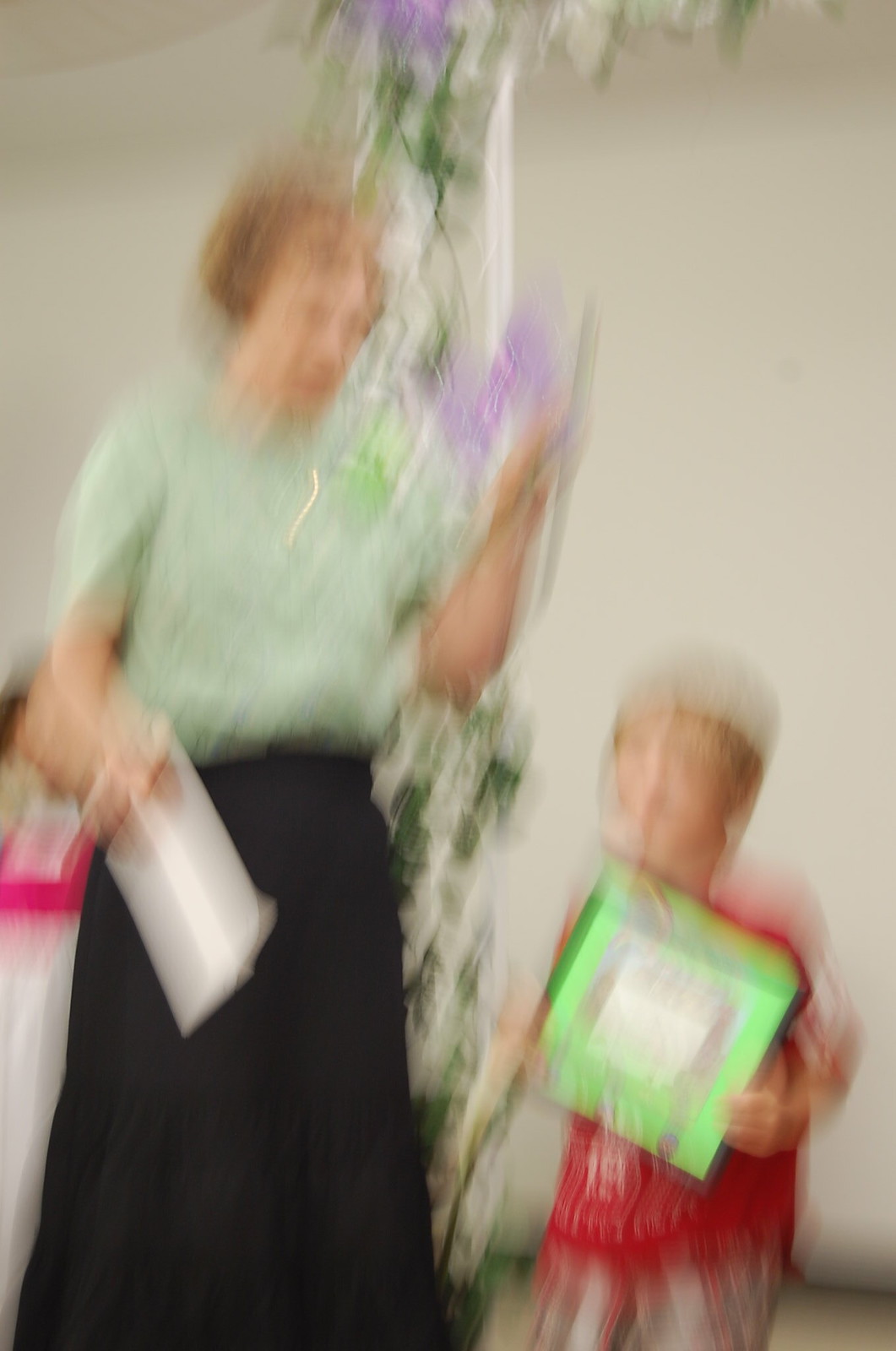In this blurry indoor photograph, a tall woman and a young boy stand side by side in front of a decorative archway adorned with green vines and occasional bunches of purple flowers. The woman, situated on the left, has short brownish-blond hair and is wearing glasses. She dons a short-sleeved light green shirt and a long black skirt. Her right hand holds a white rectangular piece of paper or an envelope, while her left arm is bent at the elbow and raised slightly. She appears to be speaking, her gaze directed towards the boy. The boy, standing to her right, has a similar hair color to the woman's and is dressed in a red t-shirt and plaid shorts containing shades of gray, red, and blue. He clutches a bright green, square-shaped object, possibly an award or certificate, that obscures much of his torso. The entire scene is somewhat blurred, suggesting the photo was taken while the camera was in motion. The backdrop features a beige wall with a white trellis archway, enhancing the composition with a touch of greenery and florals.